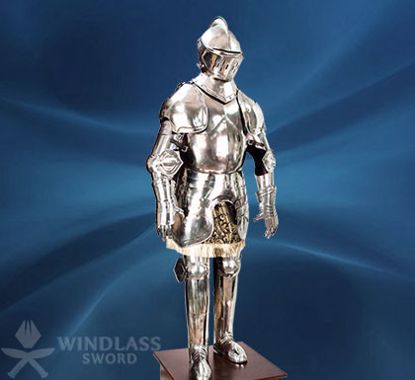The image depicts a highly detailed miniature model of a medieval knight, completely encased in polished, fully plated silver or steel armor. The knight stands on a small wooden platform against a dark blue gradient background that transitions from light to marine blue. The armor includes a helmet with narrow slits for the eyes, nose, and mouth, and features a metallic skirt around the waist. The limbs are intricately connected, with the arms strapped together using leather. This image serves as an advertisement for Windlass Sword, whose logo, a pair of cross swords with a stylized diamond above, is prominently displayed in the lower left corner along with the brand name in black caps. The overall muted tone of the image emphasizes the striking central figure of the knight.